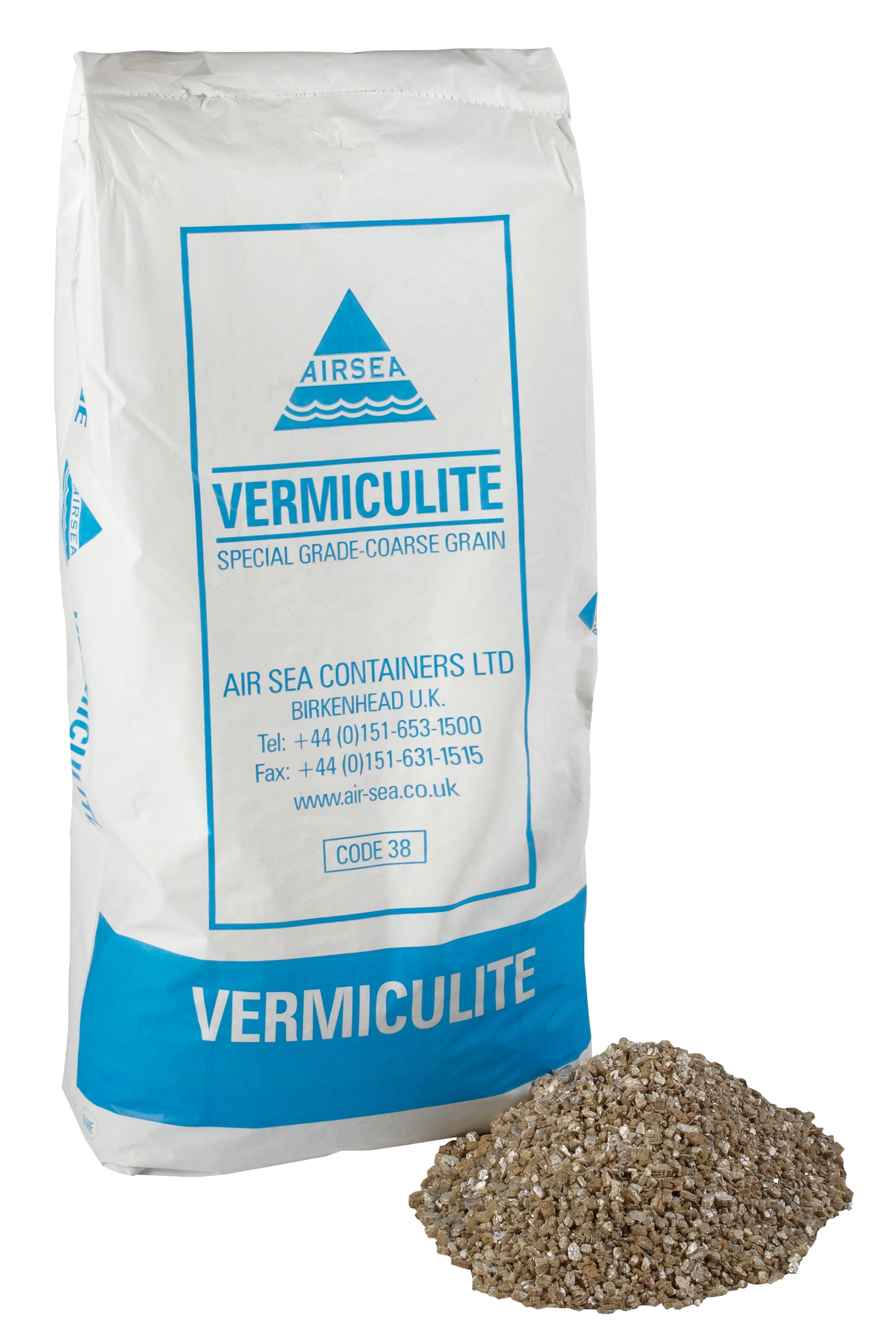The image showcases a white product package from Air C Containers Limited, prominently featuring a triangle-shaped logo at the top that reads "Air C." Below the logo, the package details its contents as "Special Grade Coarse Grain Vermiculite" and includes the address "Birkenhead, UK." Additional information such as a website "air-c.co.uk" and contact phone numbers are also visible. 

Beside the bag is a pile of coarse, brown vermiculite grains, with some lighter-colored specks interspersed. The background of the image is entirely white, providing a stark contrast that highlights the product package and the granular vermiculite. The composition emphasizes the texture and appearance of the vermiculite, making it clear that it is a coarse, sand-like material.